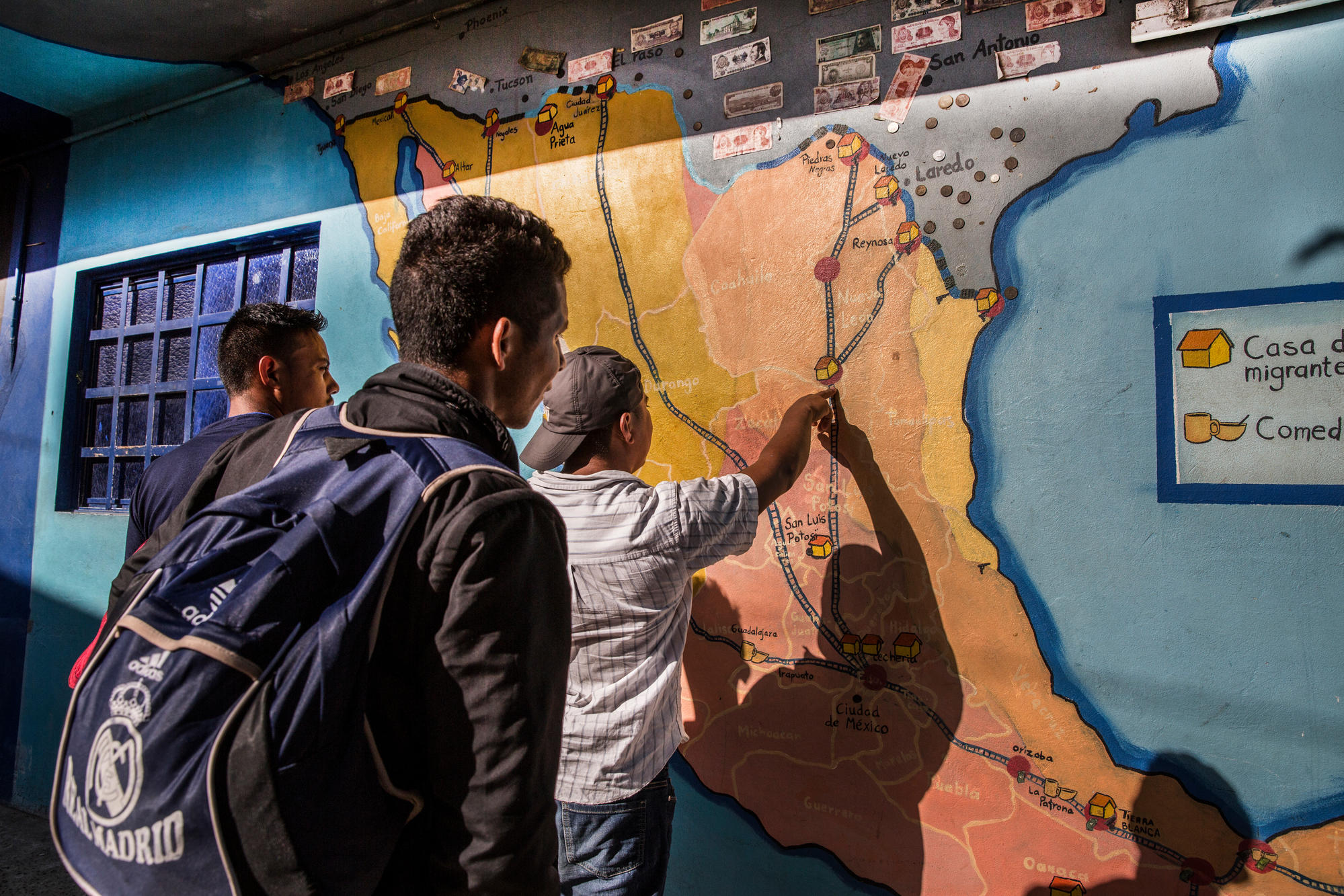In the indoor photograph, three men—two adults and one younger male—are seen in front of a wall. One man, notable for his tan skin, is wearing a warm jacket and a navy-blue Adidas backpack labeled "Madrid." The younger individual, possibly of Spanish or Central/South American descent, is dressed in a brown and cream-colored short-sleeved shirt with a collar and a backwards gray hat. He points to a wall map of Mexico, specifically highlighting a route to Texas and featuring landmarks such as "San Antonio." The map includes blue water on the right and highways marked clearly. Additionally, the wall displays paper currency and glued coins, along with labels such as "Casa Migrant" and "C-O-M-E-D" next to an image of a house and a cup with a saucer, indicating a migrant trail and essential stops for food and shelter along the border.